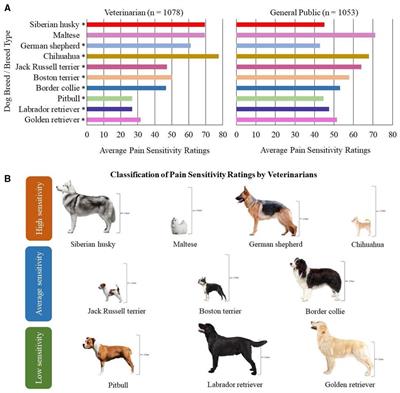The image is an intricate chart detailing pain sensitivity ratings for various dog breeds, segmented by assessments from veterinarians and the general public. At the top, there are two bar graphs with colorful bars representing different dog breeds and their respective pain sensitivity ratings. The graph labeled "Veterinarian" (N = 1078) shows ratings for breeds such as the Siberian Husky, Maltese, German Shepherd, and Chihuahua, with Huskies and Malteses having a high sensitivity rating of 70, in contrast to the general public's perception, which rates Huskies at 45 and Malteses slightly higher at around 72. The second graph, labeled "General Public" (N = 1053), mirrors this structure but shows variations in the public's perception of pain sensitivity.

Below these graphs, there's a visual classification of pain sensitivity ratings by veterinarians, organized into categories: high, average, and low sensitivity. The high sensitivity category includes breeds like Siberian Huskies, Malteses, German Shepherds, and Chihuahuas. The average sensitivity category features Jack Russell Terriers, Boston Terriers, and Border Collies. The low sensitivity category lists Pit Bulls, Labrador Retrievers, and Golden Retrievers. Each breed is depicted with a graphical representation, providing a comprehensive visual comparison of sensitivity levels among these common dog breeds.